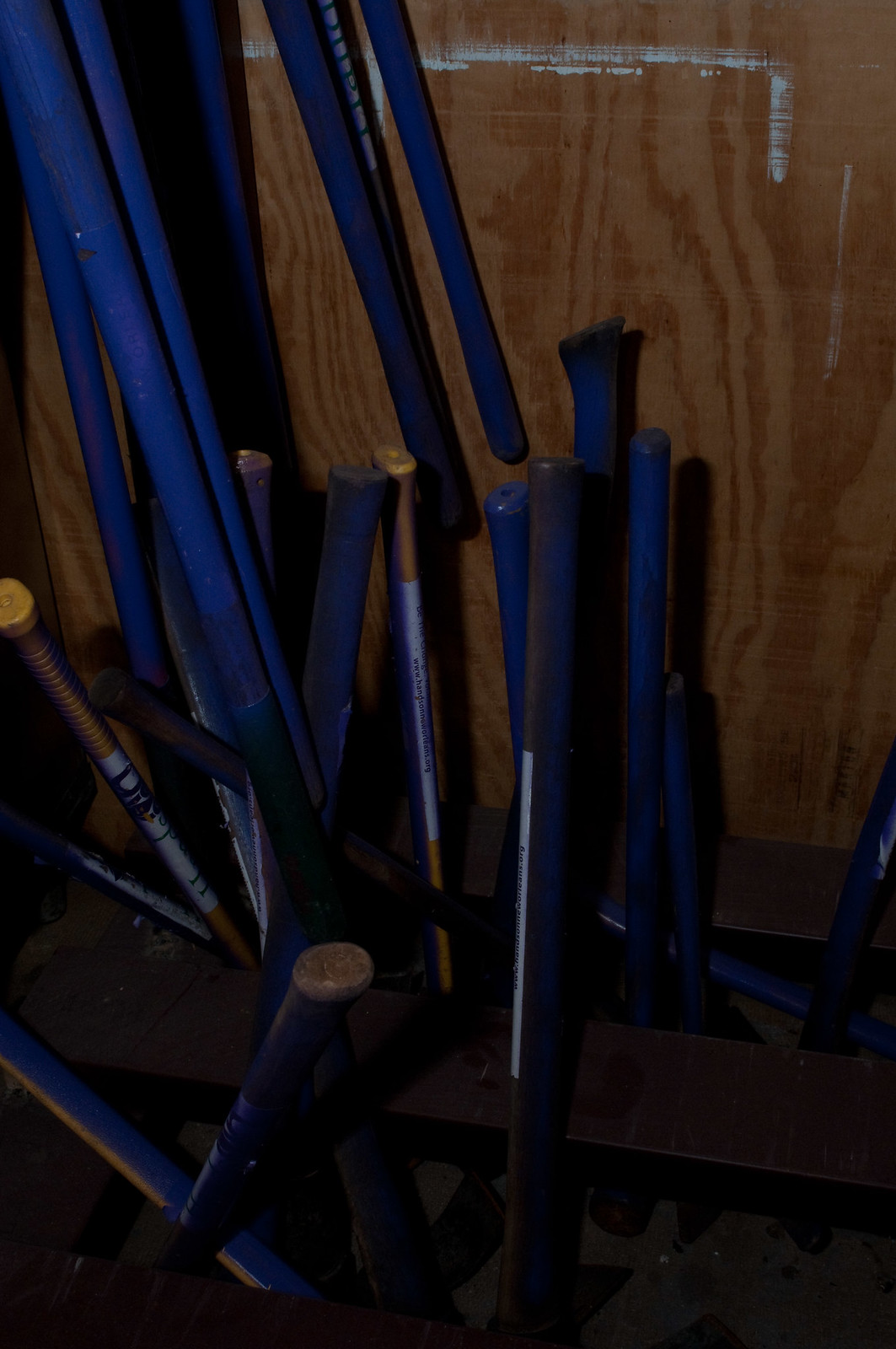The photograph depicts a dimly lit scene inside a wooden shed or room, showing a disorganized collection of blue metal tools. The front-view angle captures mostly the handles, some of which are vertical while others are leaned haphazardly against a wooden wall. The majority of the handles are painted a bright royal blue, with a few featuring orange and white stripes. Some handles end in silver, showing signs of wear as if they've been struck with a hammer. The tools appear to be resting in a roughly finished, brown wooden rack, with some lying on the ground and others standing upright or flopped over. The scene is cluttered with an assortment of these items, which seem to be for a specific purpose, possibly related to a game or task, though their exact function is unclear. The background consists of plywood, and the floor appears to be a combination of dark wood and concrete. A narrow splotch of pale blue or white paint stretches across the top of the rack. The overall disarray and poor lighting contribute to the difficulty in precisely identifying the tools.